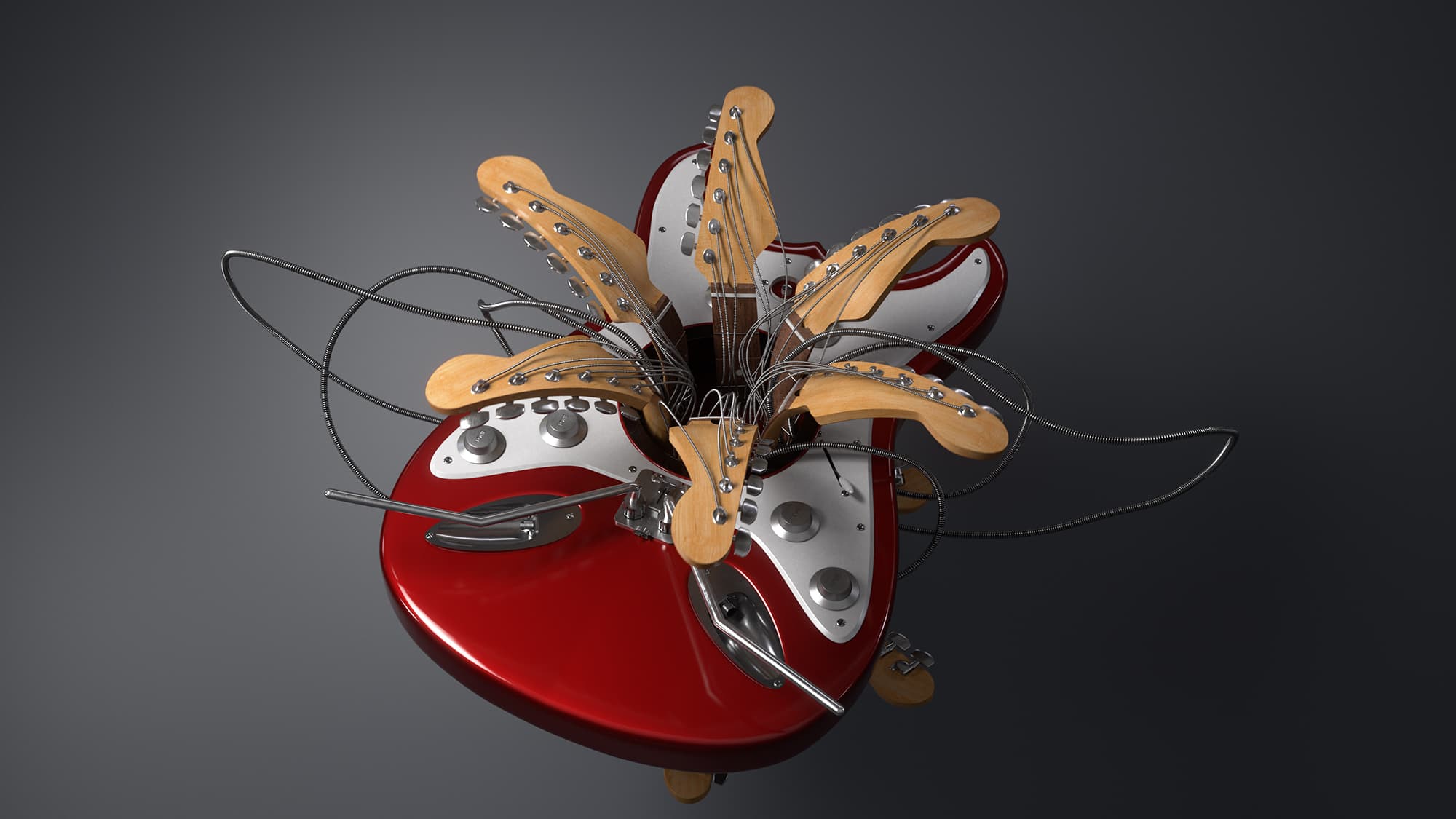The image portrays a highly abstract and detailed artistic depiction of an electric guitar. The guitar, resembling a Fender with its red body and white center, serves as the focal point. Emerging from the guitar’s central hole, traditionally the sound hole, are six necks of a guitar, their tuners creating a flower-like structure that bursts outward in a star pattern. These necks, made from light brown wood, appear to be intricately and purposefully arranged, lending a surreal and dynamic quality to the piece. Wrapped around this assembly are thick, grayish-silver wires that coil haphazardly around the guitar and its blossoming necks. Silver tuning buttons adorn both the primary guitar and the additional necks. The background of the image transitions from a light gray at the center to a dark gray at the edges, enhancing the contrast and drawing attention to the vibrant focal elements. The entire composition suggests a creative and imaginative sculpture, merging disparate guitar components into a cohesive and striking piece of art.